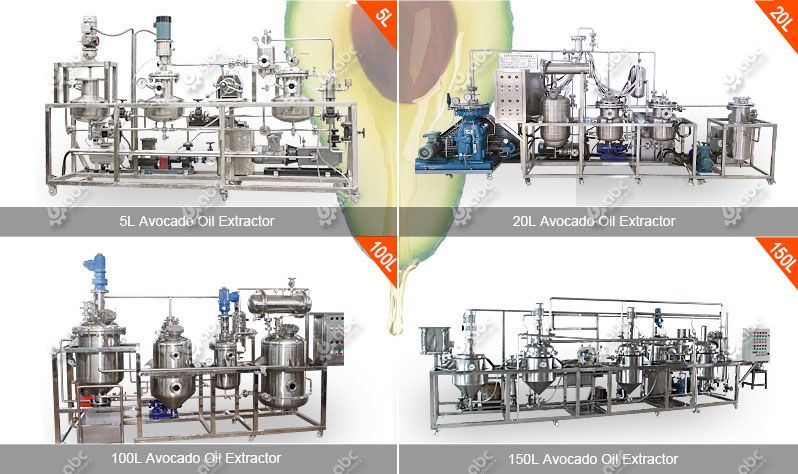The image depicts four detailed sketches or drawings of avocado oil extractors, each labeled with their respective extraction capacities. These complex machines, primarily silver in color, feature various interconnected stainless steel cylinders, pipes, and tubs. The extractors are organized as follows: the top left displays the 5L Avocado Oil Extractor, the top right is the 20L Avocado Oil Extractor, the bottom left shows the 100L Avocado Oil Extractor, and the bottom right illustrates the 150L Avocado Oil Extractor. Notably, the 20L model includes a distinctive blue section, resembling a motor, which sets it apart from the others. The extractors are sophisticated, with designs incorporating cylindrical and hourglass-shaped containers, all connected by an intricate network of tubes and pipes. Each machine is documented with a gray rectangular box indicating its capacity, enhancing the viewer's understanding of these advanced oil extraction devices.